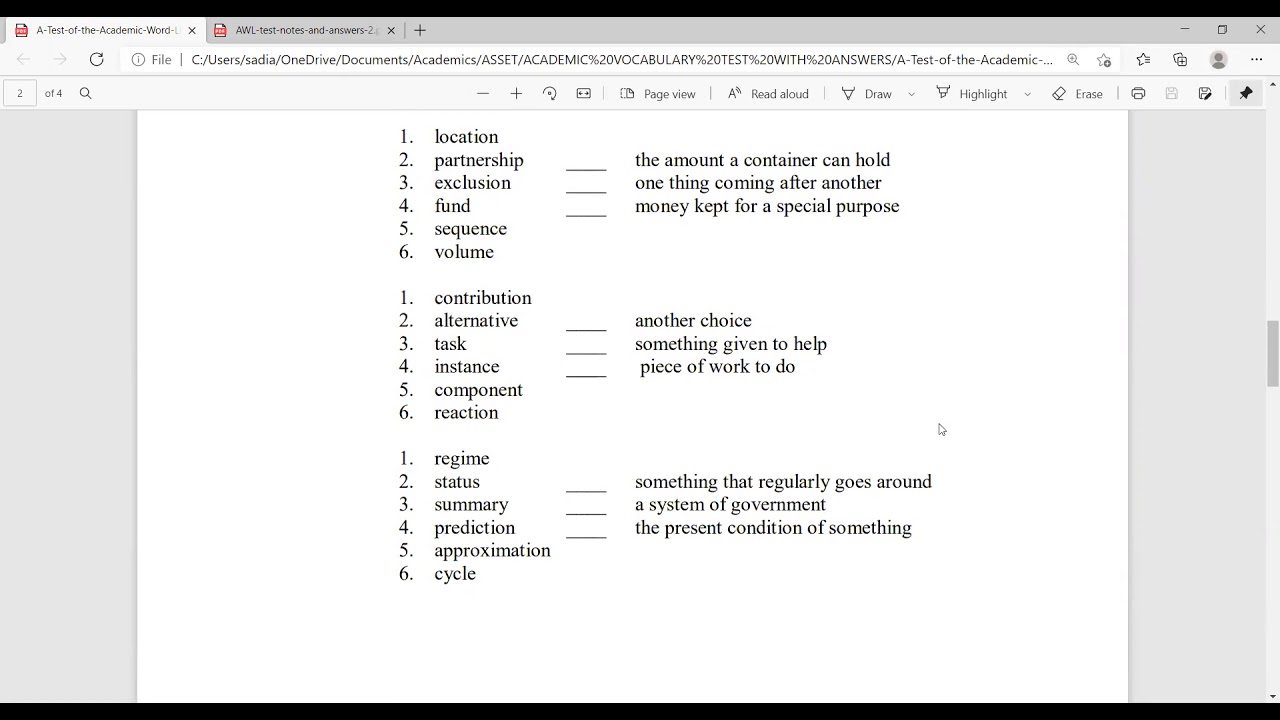This image showcases a web browser interface. The browser has two tabs open, positioned at the top left corner, both featuring identical red, white, and black icons. Beneath the tabs, the web address bar displays a lengthy URL. Central to the image is a white background, framed on both sides by vertical gray borders.

The white background contains three text sections arranged in columns, each presenting a list of terms accompanied by corresponding information. The first section lists: 1. Location, 2. Partnership, 3. Exclusions, 4. Fund, 5. Sequence, 6. Volume. The second section includes: 1. Contribution, 2. Alternative, 3. Task, 4. Instance, 5. Component, 6. Reaction. The third section features: 1. Regime, 2. Status, 3. Summary, 4. Prediction, 5. Approximation, 6. Cycle. To the right of each of these terms, detailed information is provided, elaborating on the concepts listed.